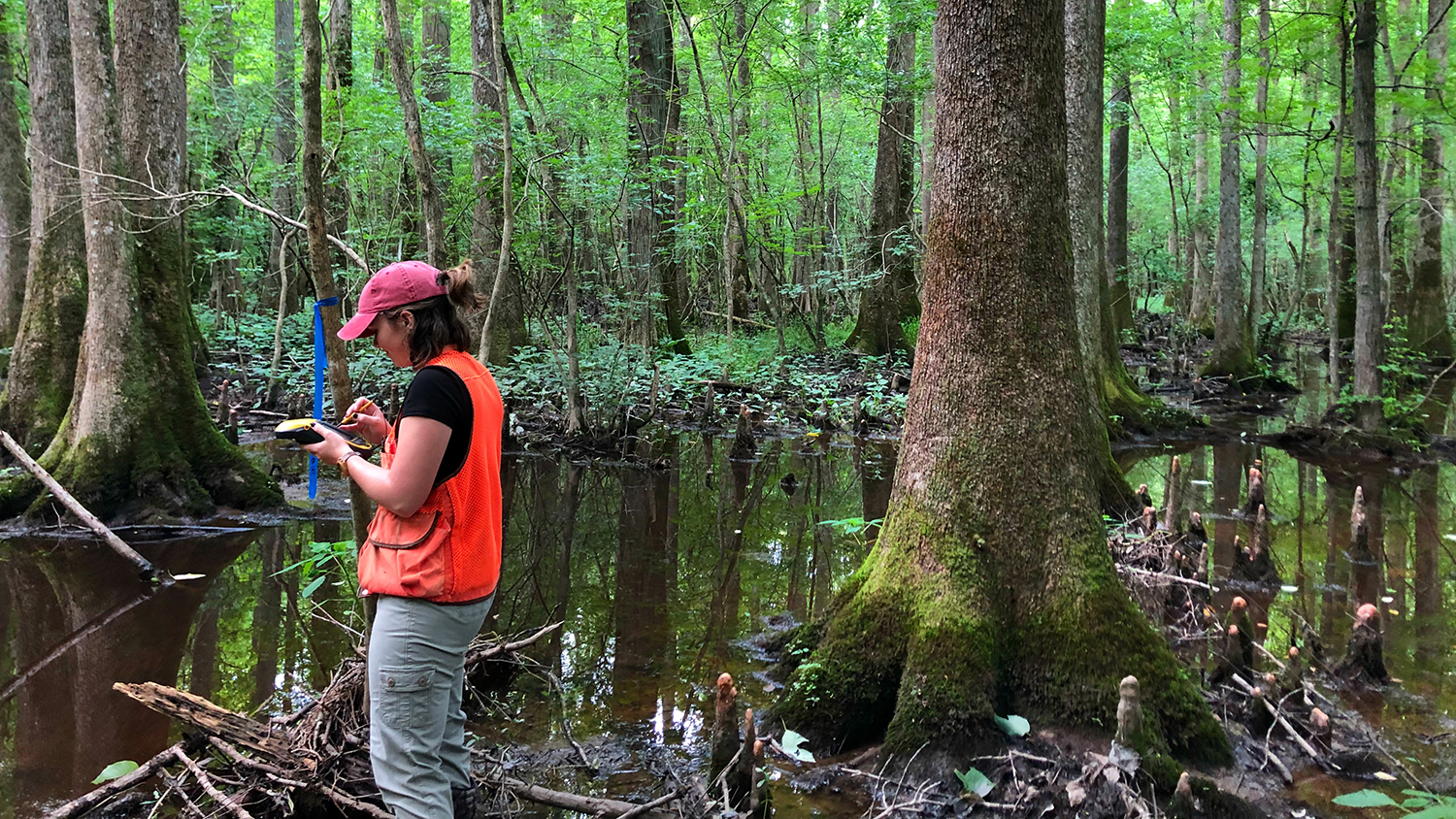In this serene swamp-like setting, a young woman stands on the left, dressed in an orange fluorescent vest over a black T-shirt, paired with light red baseball cap and gray khaki pants with large side pockets. Her hair is tied back in a ponytail, peeking out from under her cap, and she appears focused, possibly surveying the land with a tablet and pencil in hand. The scene is richly detailed with thick foliage; the ground is covered in leaves, sticks, and vines, contributing to the marshy, dense atmosphere. The still, reflective water, dark green from the tree reflections, curves around the land to the right, creating a striking backdrop. Large, moss-covered tree trunks rise from the water's edge, alongside skinnier trees that add to the forest's lush tapestry. This image perfectly captures the quiet, natural beauty and intricacy of a forest-marshland intersection.